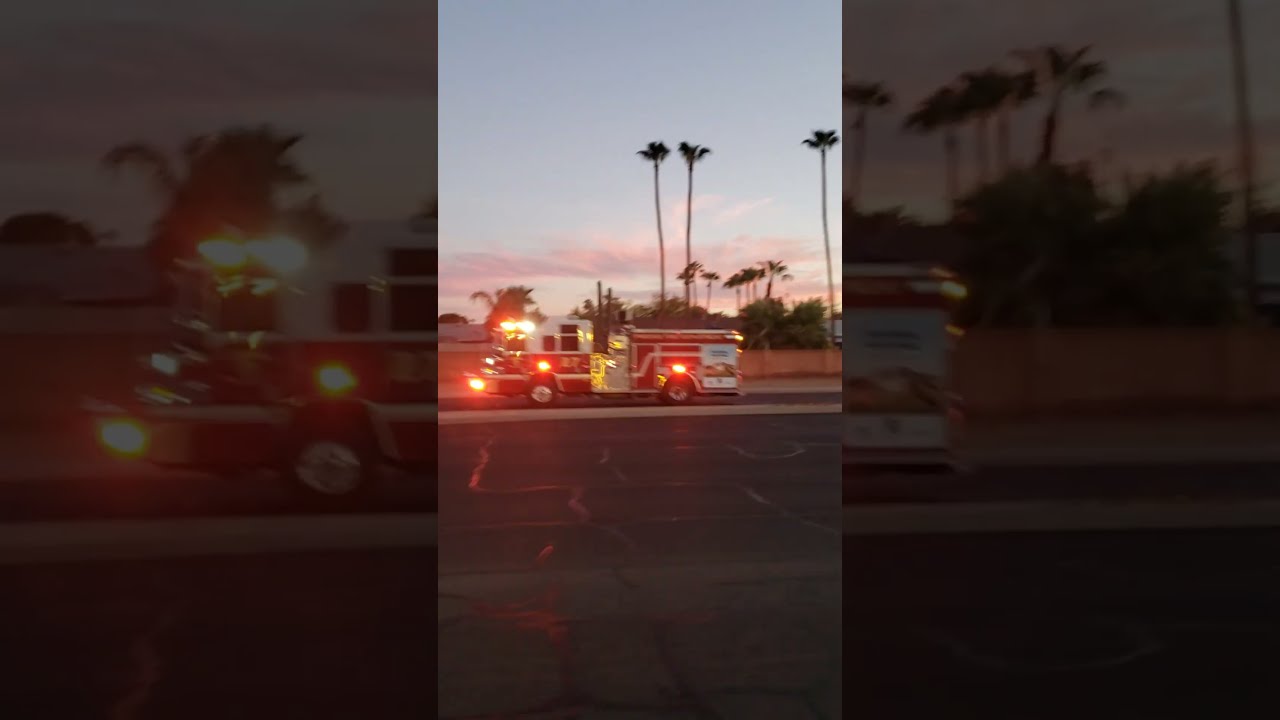The image showcases a firetruck driving down a road surrounded by a lush landscape characterized by tall and short palm trees, indicating a tropical or southern location. Dominating the center of the composition, the red and white firetruck flashes its lights as it speeds toward an emergency, clearly visible from both the front and the sides. The visual is taken at dusk, evidenced by the bluish sky transitioning into hues of pink and purple as the sun sets. The scene is set against a mixed backdrop of dark and bright tones; the central strip of the image is vividly in focus and well-lit, while the left and right sections are notably darker. The bottom half of the image features dark gray pavement, contrasting with the lighter, partly cloudy sky above. This wide rectangular image also includes close-up sections on each side, which are shaded darker but emphasize the middle shot. The colors span black, white, yellow, orange, red, green, blue, purple, and pink, adding to the vibrant yet dramatic atmosphere.